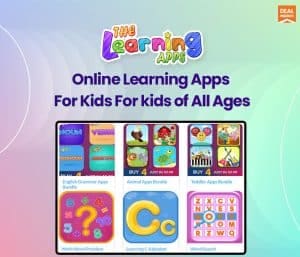The background of the image features a vibrant gradient of colors: starting with a soft pink in the bottom left corner, transitioning to blue in the top left, then morphing into a light yellowish-green in the top right, and finally blending into a blue-green in the bottom right.

At the very top center of the image, the word "the" is displayed in a small, orange font, positioned above and partially overlapping the word "Learning." In "Learning," the first letter, "L," is capitalized and colored purple. Following this, the letters are a rainbow of colors: a green "e," a red "a," a blue "r," a fuchsia "n," a yellow "i" with a star dot, an orange "n," and a blue "g." Adjacent to the bottom right of "Learning," the word "APPS" appears in bold, all-capital letters in green font.

Beneath "APPS," a line of descriptive text in dark blue font reads, "Online learning apps for kids of all ages."

At the bottom of the image is a rectangular area containing six squares, each representing different educational games or apps available for learning.